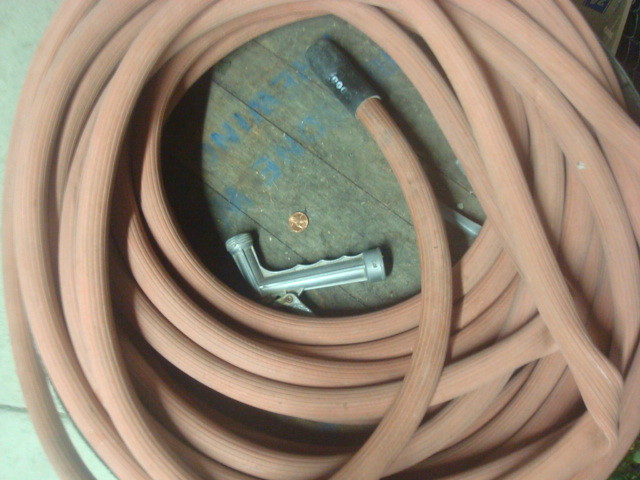The photograph captures a tan-colored water hose coiled up on an old, weathered wooden floor. The coiled hose features a black rubber section about midway and is kinked towards the right corner. On the floor within the coil, there is a shiny bronze penny, and a detachable hand-held sprayer lies nearby, which is metallic gray in color. The sprayer, designed to attach to the hose for directing water flow, rests towards the bottom of the image. There are faded blue words on the wooden planks, though they are too blurry to discern clearly.